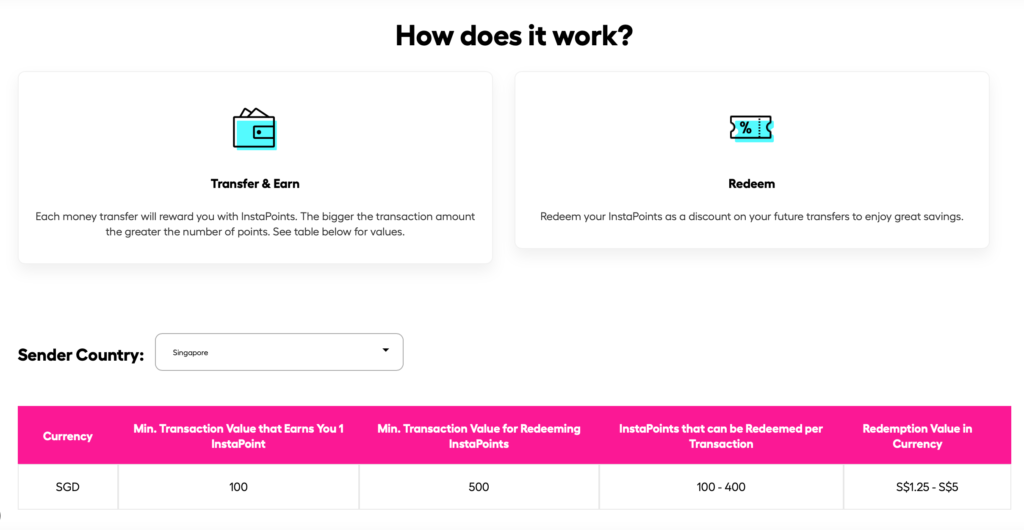This image is a screenshot of a website page related to a financial service. The background is light gray with black text. At the top of the page, a header reads, "How Does It Work?" Below the header, the content is organized into two columns titled "Earn and Transfer" and "Redeem."

In the "Earn and Transfer" column, the text explains that each money transfer rewards the user with "Instapoints." The number of Instapoints earned increases with the transaction amount. A table below provides specific values.

In the "Redeem" column on the right, it details how users can redeem their Instapoints for discounts on future transfers, offering significant savings. There's a section labeled "Sender Country" that includes a dropdown menu currently set to Singapore.

A table underneath lists detailed information:
- **Currency**: SGD (Singapore Dollar)
- **Minimum transaction value that earns you one Instapoint**: 100 SGD
- **Minimum transaction value for redeeming Instapoints**: 500 SGD
- **Instapoints that can be redeemed per transaction**: 1 to 400
- **Redemption value in currency**: $1.25 to $5 SGD

The page is minimalist, with no additional significant content.